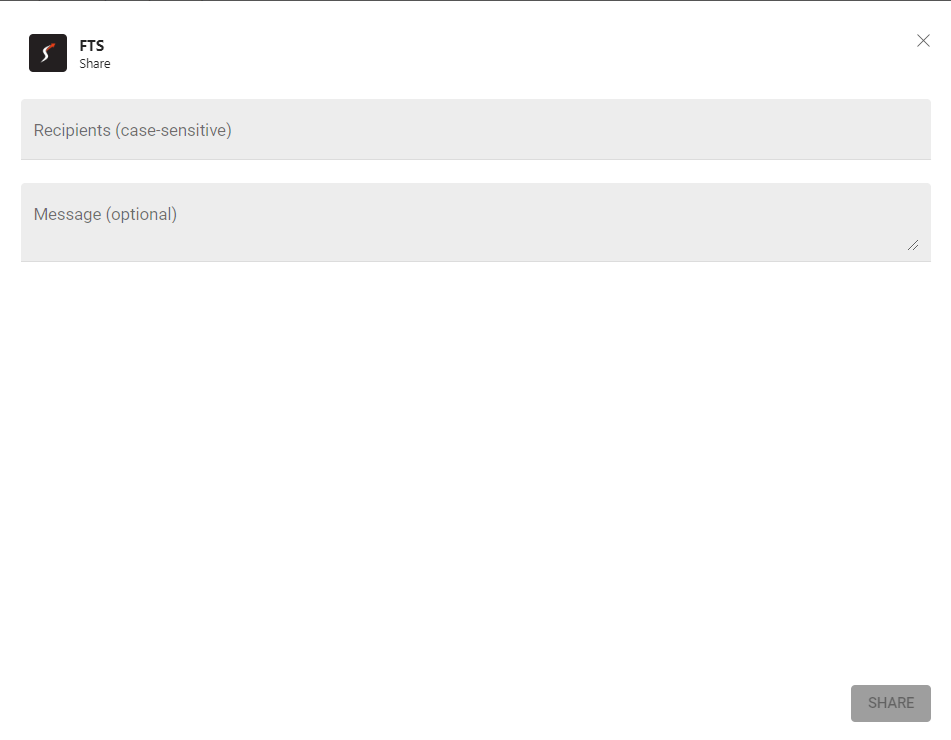The image displays a straightforward and minimalistic interface for a message-sharing platform named "FTS Share." In the top-left corner, the logo is prominently featured—a black square with a stylized white 'S' inside it, accompanied by the text "FTS Share." Below the logo, there are two main input fields. The first is a large, rectangular gray box labeled "Recipients" with a note in parentheses indicating "Case Sensitive." Beneath this, there is a smaller input box labeled "Message" with "Optional" in parentheses. At the bottom right of the screen, there's a gray "Share" button, indicating the user can initiate the sharing process by clicking it. The page maintains a clean and uncluttered design, focusing attention on the essential elements required for sharing messages.